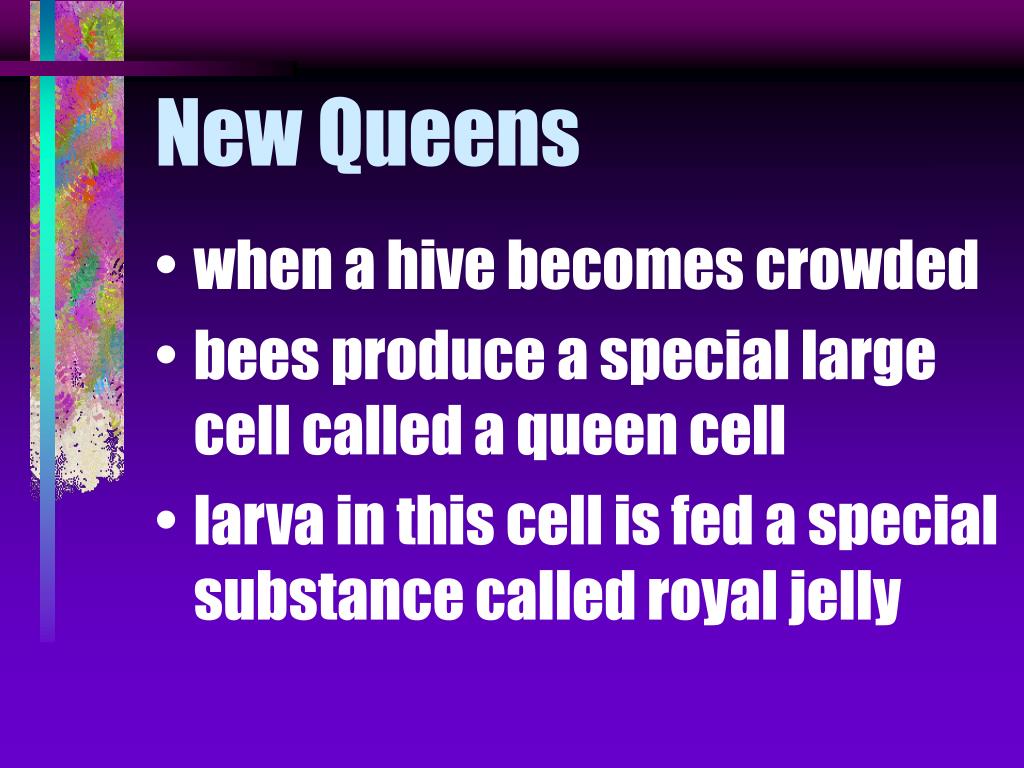This image features a detailed slide from a presentation, with a visually striking background that transitions from a medium purple to dark purple, and then fades to magenta-violet at the top. The left side of the slide is adorned with a narrow, multicolored decorative banner resembling a tie-dye or paint splatter pattern that occupies about 10% of the width, adding a vibrant accent to the design. The banner includes blotches of various colors, predominantly purple and blue.

At the very top of the slide, the title "New Queens" is prominently displayed in a very light blue font. Below the title, three bullet points are listed in white text:
1. "When a hive becomes crowded."
2. "Bees produce a special large cell called a queen cell."
3. "Larvae in this cell is fed a special substance called royal jelly."

This succinct and informative slide utilizes a harmonious color gradient and creative design elements to maintain visual appeal while effectively conveying key points about the behavior and biology of bees.